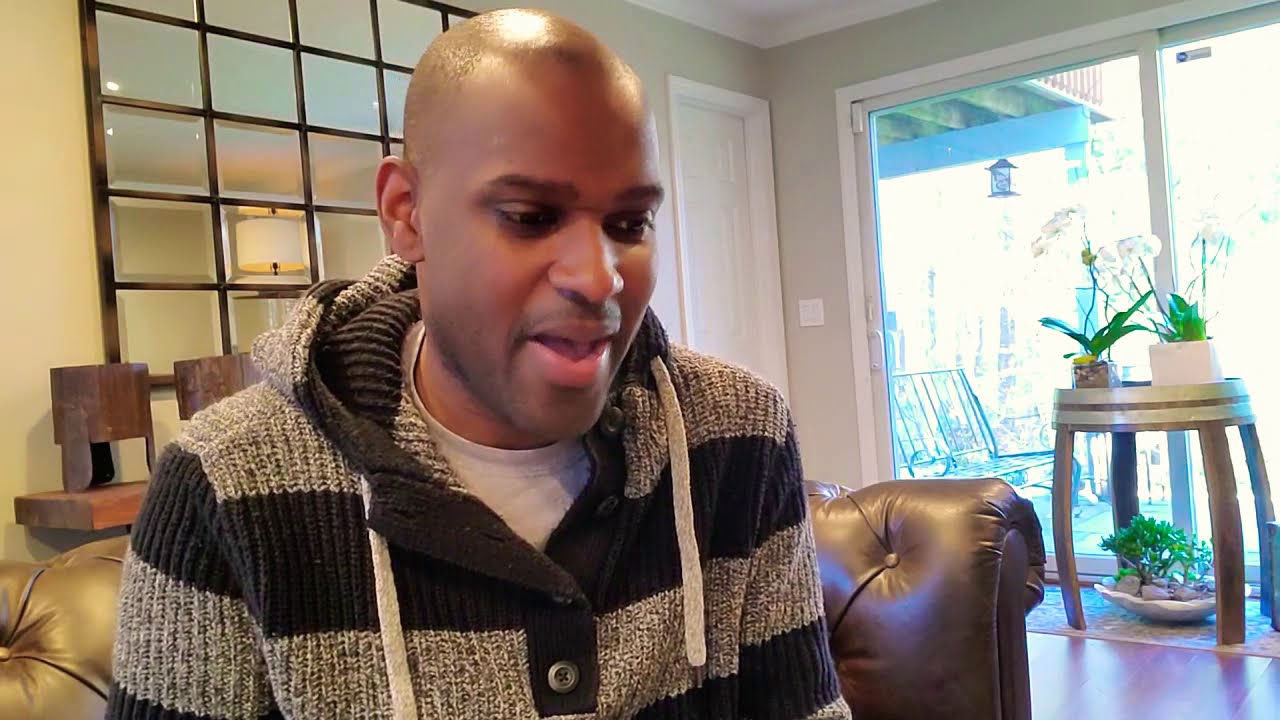This landscape photograph captures a dark-skinned man, possibly in his young adulthood, seated on a luxurious brown leather couch adorned with tufted buttons. The man has a nearly shaved head with a light stubble of hair and no notable facial hair. His expression is one of surprise and elation, his gaze directed slightly downward, perhaps focused on a television or some other point of interest.

He wears a stylish ensemble comprising a gray and black striped wool hoodie with a white t-shirt peeking out from underneath. The couch is positioned in a well-lit living room featuring hardwood floors, pale light green walls, and various sophisticated decor elements. Behind the couch, on the right side of the image, there is a set of sliding glass doors that lead to a bright, sunny backyard. The light pouring in suggests that it's a clear day outside.

Next to the sliding doors stands a small elegant table with curved legs, holding two plants with lush green leaves and a bonsai tree underneath. To the left of the couch, behind the man, is a distinctive mirror framed in brown and black wood with a lattice-like crosswork pattern, adding a touch of sophistication to the room. The mirror reflects a lamp post, indicating another room but blurring whether it's a mirror or a window. Adjacent to the sliding doors, there's a white doorway which likely leads to another part of the house.

The backyard visible through the glass doors features a bird feeder and a bench, enhancing the cozy and inviting atmosphere of this living space.